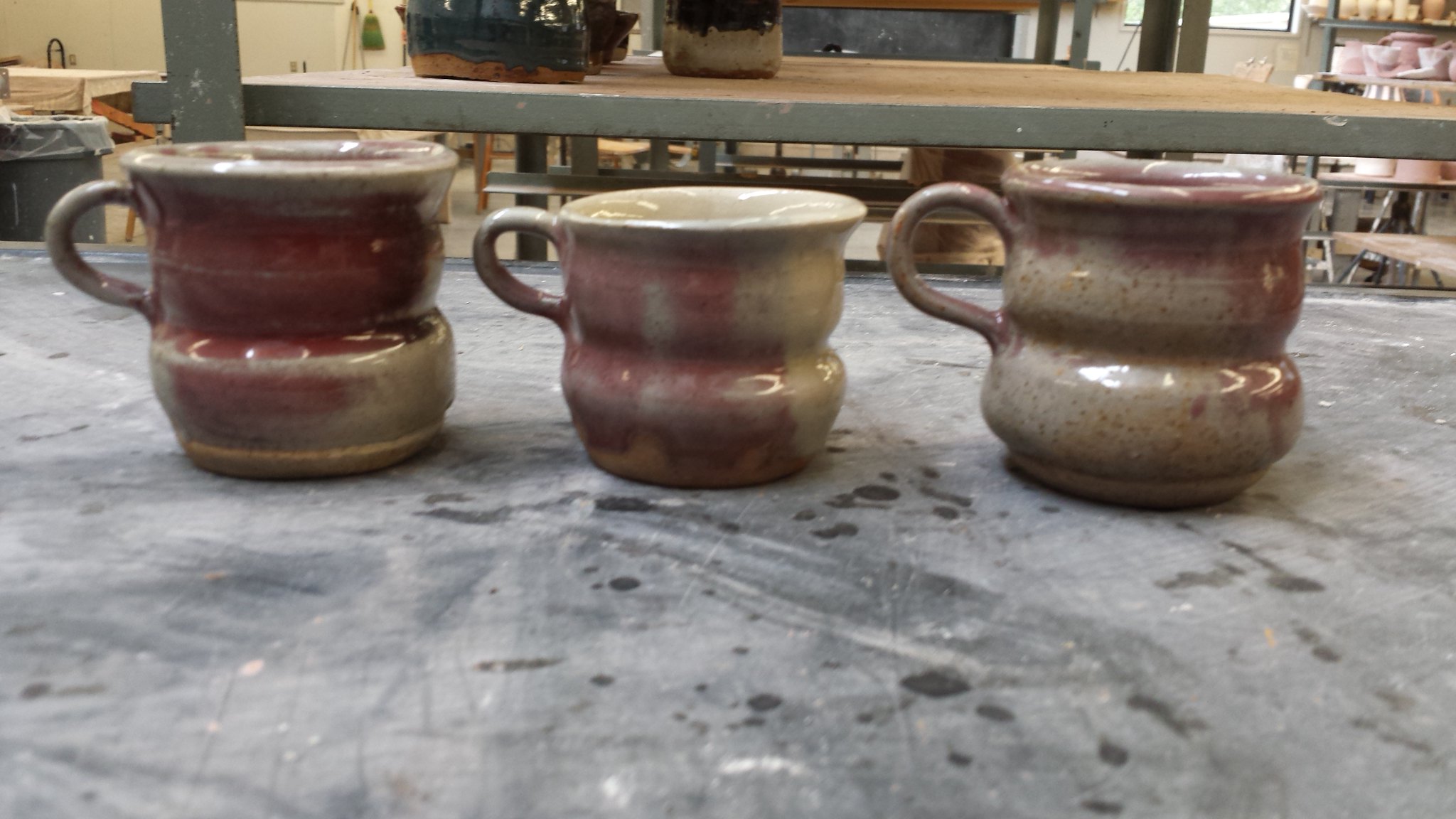In this detailed image, three handcrafted ceramic mugs are the primary focus, each positioned front-facing on a gray, dust-covered table. The gray table occupies the frame from the bottom up to about two-thirds of the image. The mugs are arranged from left to right, with the leftmost mug being slightly larger and taller. This mug features a handle facing to the left and displays a grayish rim, a red middle section, and a mixed gray-red base with a brownish lip.

The middle mug is shorter and comprises two distinct layers: a gray handle pointing left, with its body transitioning from red on the left and center to light brown on the right. The rightmost mug resembles the first with its handle also facing left. It is predominantly gray on the left two-thirds, transitioning into red towards the end.

In the background, a brown table with green metal supports is visible; atop it, a mysterious object rests indistinctly on the left side. Additionally, a gray trash can and a piece of brown wood or station are positioned to the left above this table. Further back, shelves filled with various pieces of pottery, both finished and unfinished, suggest that this scene is set in a ceramic studio.